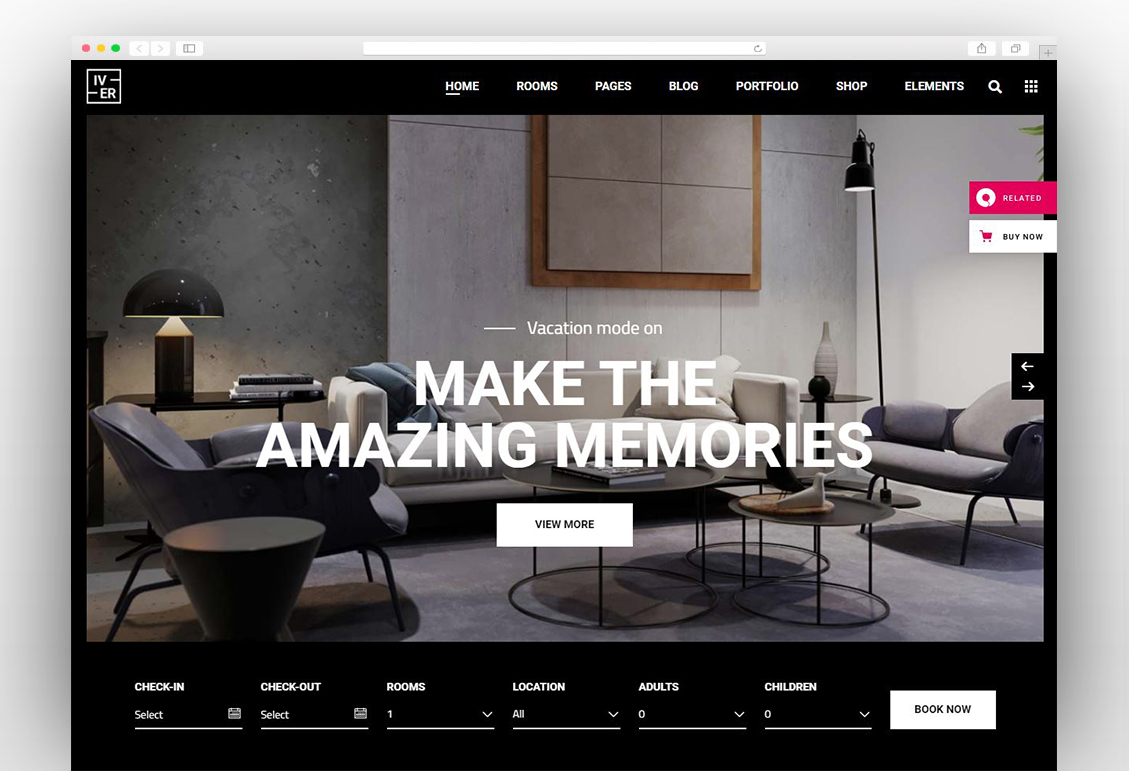The website, displayed on a Mac computer with a light gray border, features a dark-themed design with a predominantly black background. The header includes white navigational text that reads: "Home," "Rooms," "Pages," "Blog," "Portfolio," "Shop," and "Elements." Adjacent to these links is a search bar, and a dotted box is also visible on the page.

The central image showcases a cozy living room setting accompanied by text that encourages, "Make the vacation mode on, make the amazing memories." To the left of this image, a prominent pink box with a white circle contains the word "Related." Below this, a white box with black writing reads "Buy Now," accompanied by a small pink shopping cart icon.

The living room pictured includes end tables, coffee tables, and two lamps. The decor is minimalistic and somewhat bland, featuring only a few decorations. Below the motivational text, "Make the amazing memories," there is an option that says "View More."

Towards the bottom of the page, several interactive fields are available for making reservations, including "Check In," "Check Out," "Rooms," "Location," "Adults," "Children," and a "Book Now" button, suggesting the website's focus on vacation and booking services.